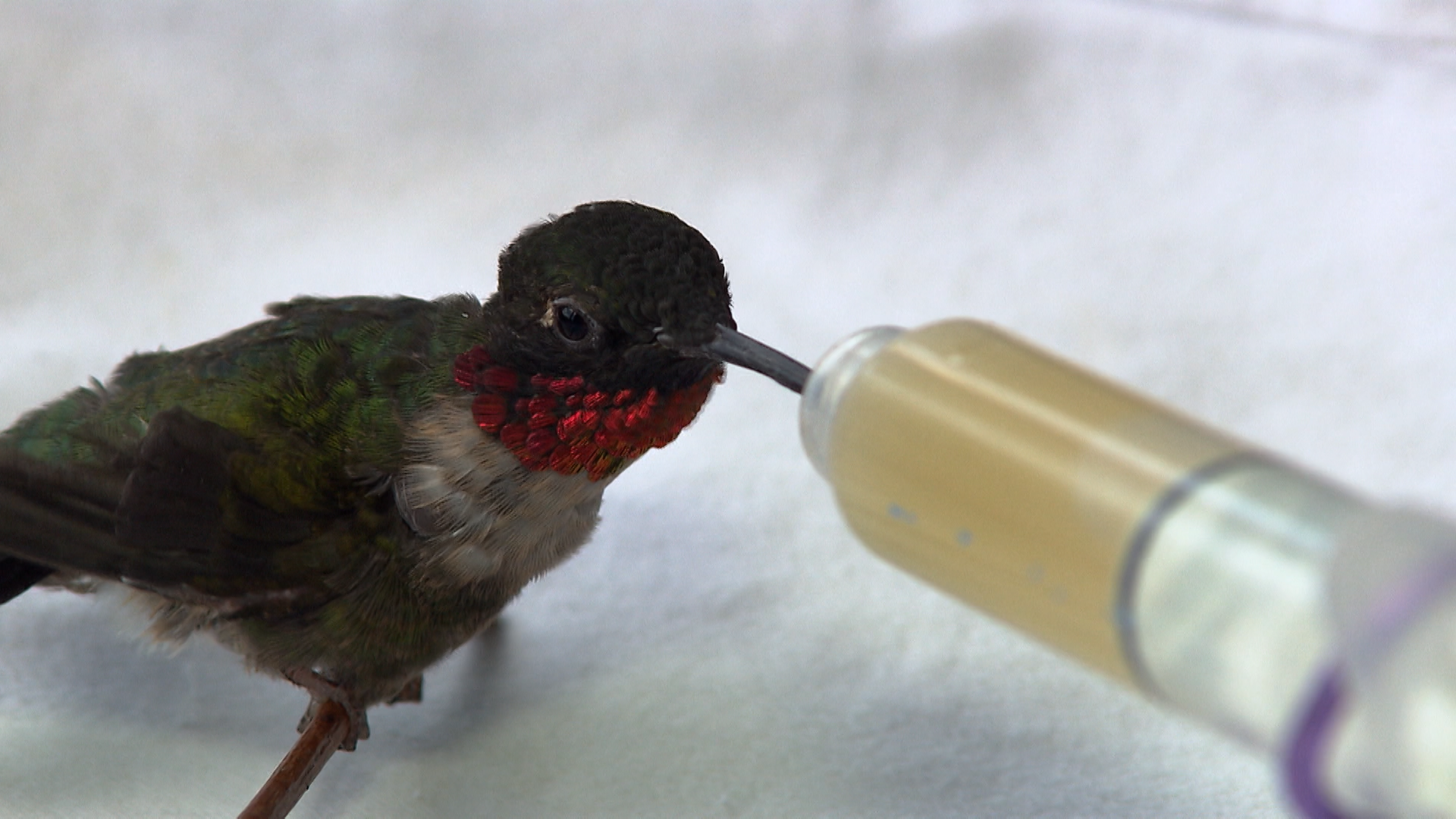This detailed color photograph captures a small, bedraggled hummingbird perched on a slender twig, facing to the right. The bird, with its ruffled feathers, sports a dark green coat, a bright red iridescent throat, a white chest, and a black-capped head. Its slender black beak is inserted into a syringe that contains a golden, amber-colored liquid, likely nectar or syrup, filling about three-quarters of the syringe. The backdrop consists of a white material, possibly cotton batting or a towel, emphasizing the bird's vibrant plumage and the feeding process. The setting appears clinical, with no visible people, other animals, structures, or mechanical objects, focusing solely on the hummingbird's delicate interaction with the syringe.